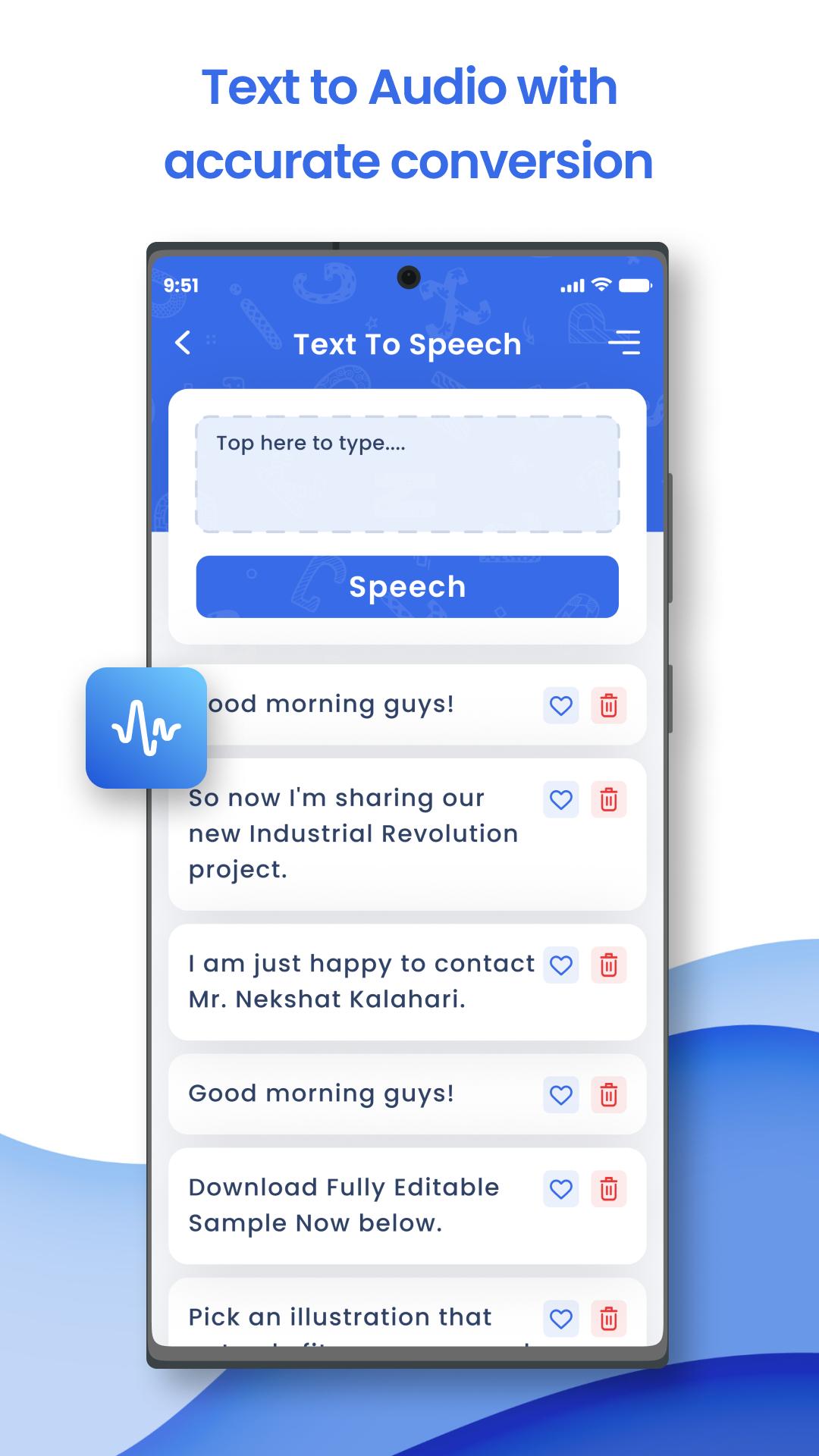This image features a screenshot set against a clean white background occupying the top two-thirds, while the bottom third showcases serene ocean waves in a gradient of light blue, medium blue, and dark blue. Dominating the top center is the large blue text that reads "Text to Audio with Accurate Conversation." 

Central to the image is a black cell phone, prominently displayed, featuring two side buttons on its right edge. The phone's screen, captured in the screenshot, reveals a time of 9:51 AM in small white text at the upper left corner of the header. The top right corner displays essential status icons in white: fully connected Wi-Fi, a completely charged battery, and maximum cellular signal bars.

The center of the phone screen is highlighted by large white text that boldly states "Text to Speech." Directly beneath this, a blue interactive text box invites the user to "Tap here to type." Below this text box, a prominent blue action button labeled "Speech" in white text beckons the user to initiate the text-to-speech function.